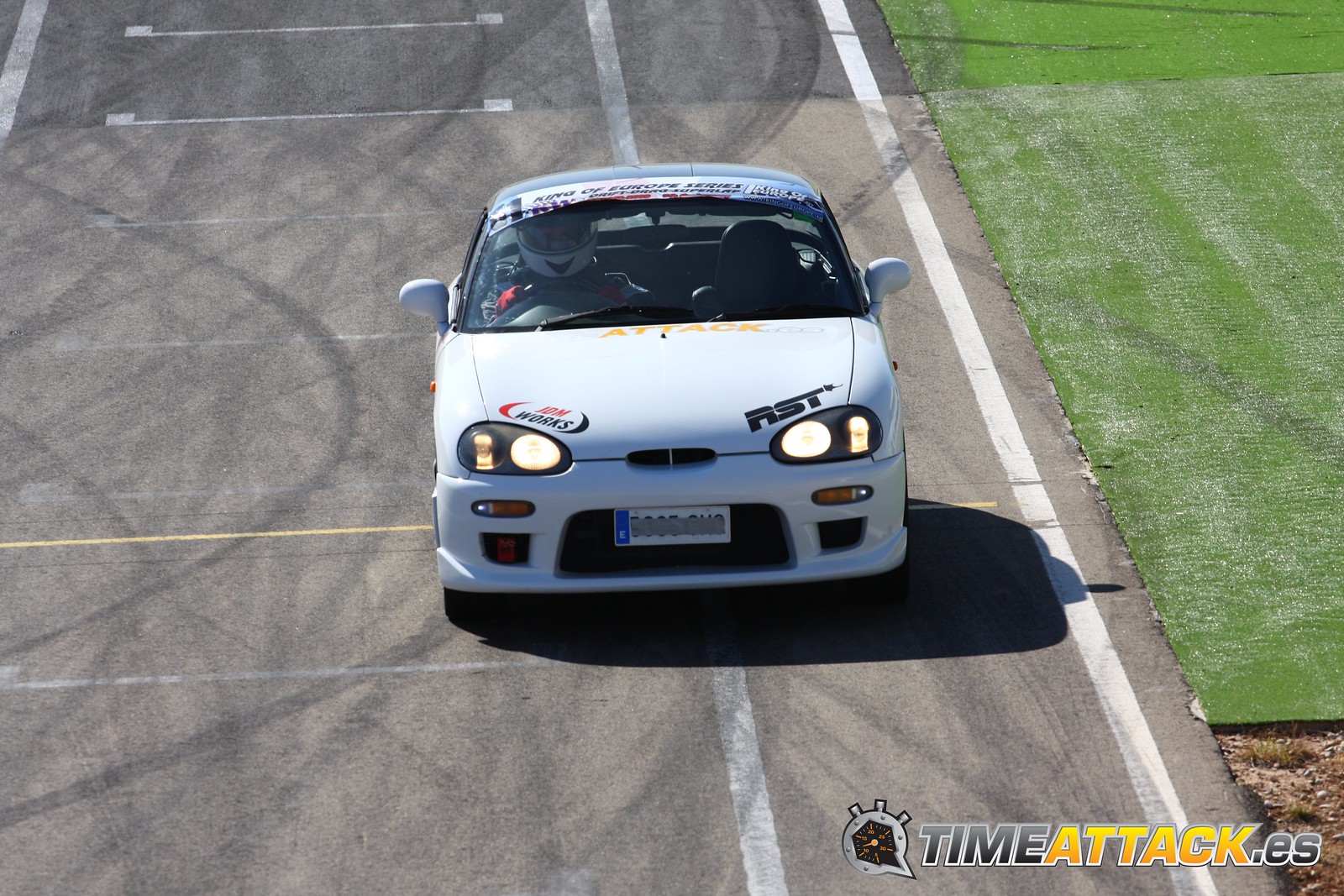This is a high-angle, overhead photograph of a white race car, prominently showing the front and top but excluding the sides and back. The vehicle, which is either a sedan or a two-door car, is adorned with multiple logos in blue, red, and yellow. The top of the car displays a banner reading "King of Europe Series," while the front hood showcases logos for "IBM Works" on the left and "RST" on the right. The car's headlights are on, and it has a front license plate in white, blue, and black. It is parked on an asphalt road marked with white lines, and to the right of the car lies a grass field, along with a small area of mulch, dirt, or weeds visible in the lower right-hand corner. In the very bottom right-hand corner of the image, there is a logo with black, white, and yellow text that reads "timeattack.es," accompanied by a small speedometer graphic. Inside the car, visible through the window, is the driver, dressed in a red driving suit and wearing a white helmet with a clear visor and a distinctive V shape around the mouth area.